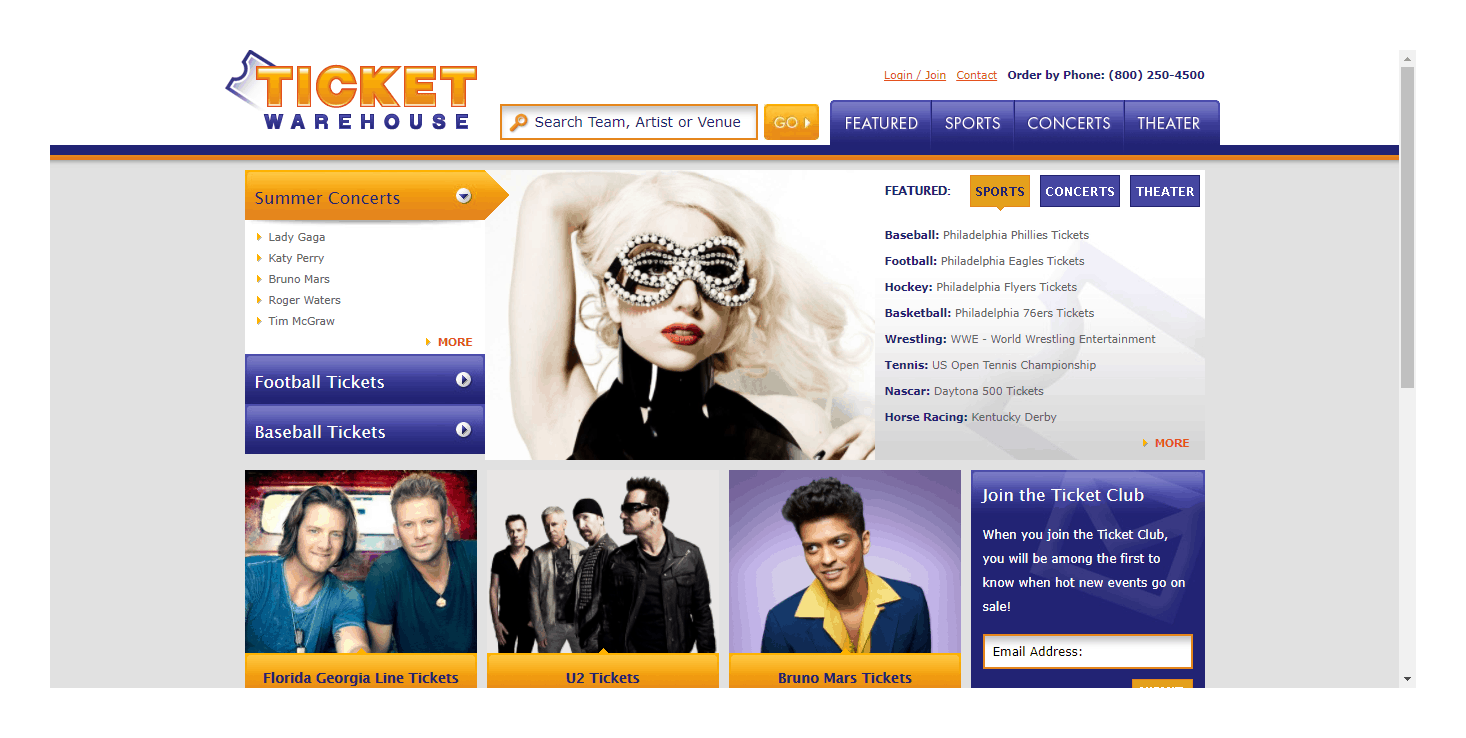The homepage of the Ticket Warehouse website is depicted in the image. The word "Ticket" is prominently displayed in vibrant orange text, while "Warehouse" is in bold blue lettering. At the top of the page, there is a search bar with the placeholder text "Search Team, Artist, or Venue" written in blue, accompanied by an orange magnifying glass icon. Next to the search bar is an orange button with the word "Go" in white. Below this are the menu options "Featured," "Sports," "Concerts," and "Theater" in white text.

Central to the page is a striking photograph of Lady Gaga, adorned with bright red lipstick and multiple pairs of sunglasses embellished with pearls. A list of summer concerts is displayed in black text, featuring high-profile artists such as Lady Gaga, Katy Perry, Bruno Mars, and Tim McGraw. 

Additionally, an image of Florida Georgia Line is shown, with the two band members seated side by side; one is in a light blue shirt and the other in a dark blue shirt. Next to them is a picture of Bruno Mars sporting a blue suit over a yellow shirt. Beneath this image is an orange bar that reads "Bruno Mars Tickets" in blue text, with a clickable red link saying "More" for additional information.